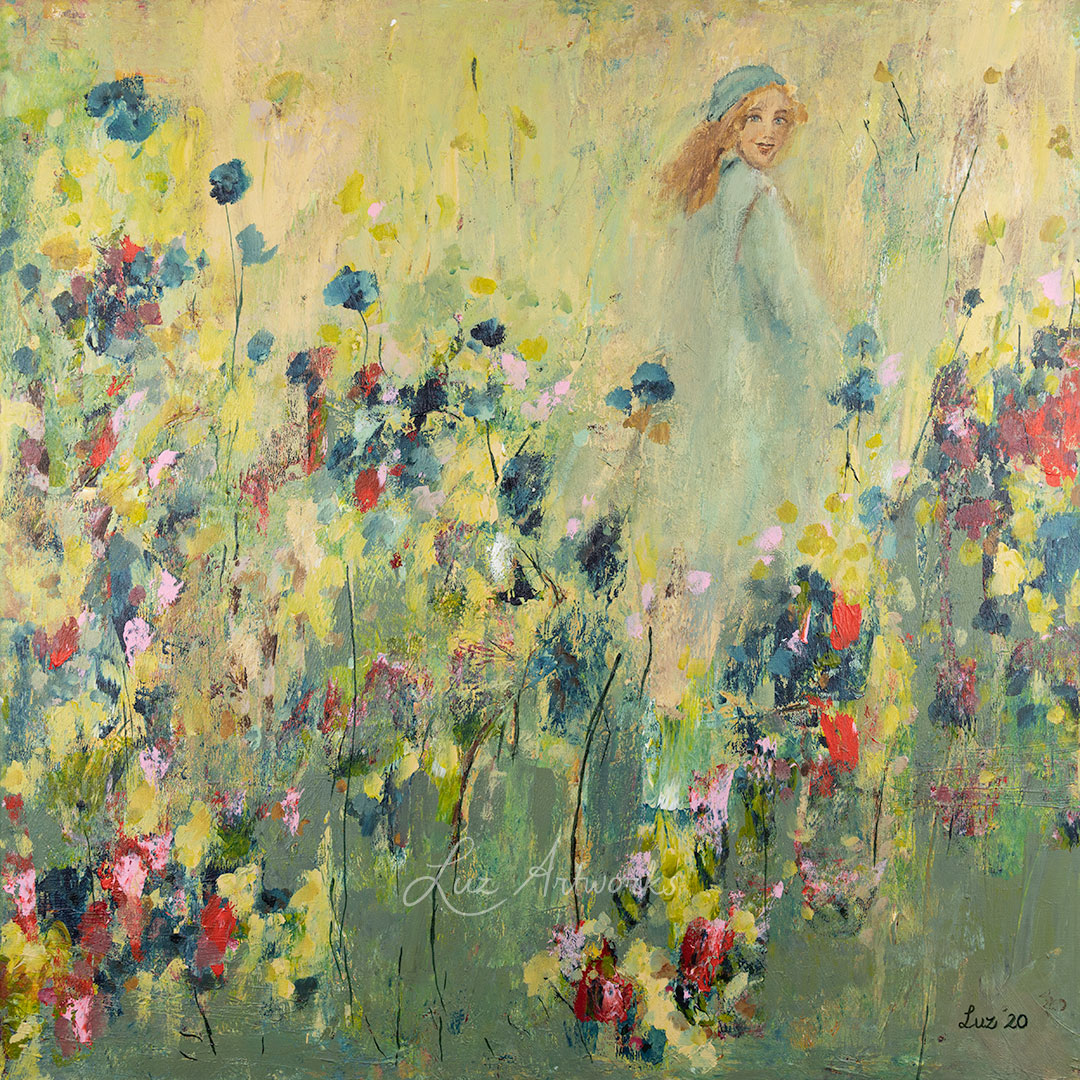The painting, an oil artwork by Luz, signed “Luz 20” in the lower right corner, is an impressionistic depiction of a woman standing in a vibrant flower meadow. The painting is square-shaped and features loose, splotchy representations of flowers in various shades of red, blue, white, yellow, and purple. The flowers cover the field from a gray-green base at the bottom to lighter white and golden hues towards the top. The central figure is a young white woman with long blonde hair, though one description mentions light brown hair, standing with her back to the viewer but with her head turned to face the audience. She wears a light blue jacket extending down to her covered knees, paired with a blue cap or bandana. The woman's attire blends harmoniously with the impressionistic floral surroundings, adding to the ethereal quality of the scene.